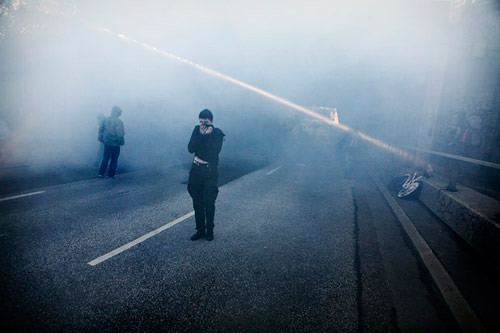The image depicts a foggy night scene on a deserted, three-lane road enveloped in smoke or fog, making visibility poor beyond a certain point. Central to the scene is a man in all black, with short black hair, standing nearest to the camera. He has both hands raised, covering his nose and mouth with his shirt. Nearby, two other figures are visible standing further down the road with their backs towards the camera. One of them is on the left, wearing a bulky jacket with its hood up and dark pants, and the other, possibly another man, stands on the right side of the road, barely discernible in the haze. A single ray of sunlight pierces the smoky scene from the upper left to the mid-right side. The white lines of the road are visible up to the point where the smoke starts to obscure everything. An outline of a vehicle emerges faintly in the background, suggesting a possible connection to the smoke or fog. A bike leans against a high curb on the right side of the image, adding to the eerie, abandoned atmosphere.